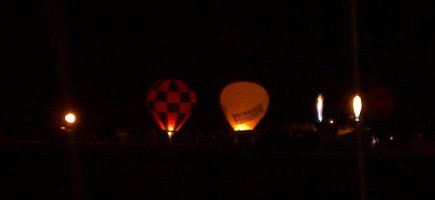In this dim, nighttime photo, we see the preparation and inflation of multiple hot air balloons from a distance, set against a nearly black sky. The focus is soft, lending a dreamlike quality to the scene. To the right, bright spots suggest the flames from gas torches, illuminating the setup process even though the balloons themselves aren't fully visible. Two hot air balloons are partially inflated: one features a black and yellow checkerboard pattern, while the other, also in black and yellow, displays a graphic or text on its side. Both balloons have a golden glow emanating from their bases, indicating the presence of the burners heating the air inside. Additional torches on the left are actively inflating other balloons, though these are not yet visible. The varied intensity of the flames and lights highlights different stages of inflation and preparation for ascent. The entire scene is framed against a near-black background, capturing the quiet, methodical beauty of a night-time balloon launch preparation.